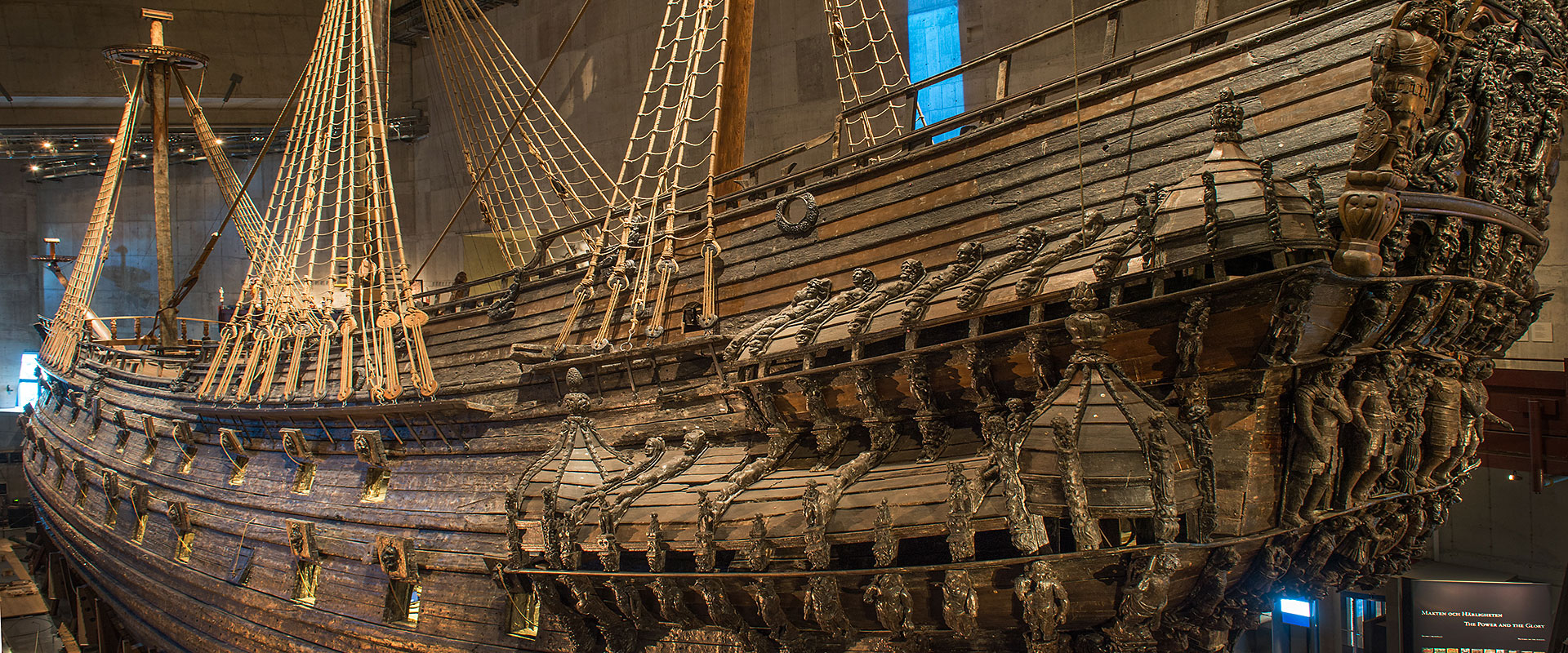The image is a detailed close-up of what appears to be an old wooden pirate ship, likely on display in a museum. Captured at an angle from the left-rear side, the photograph showcases the intricate craftsmanship of the vessel, including rows of windows that likely served as cannon ports. The ship, devoid of its sails, features numerous ropes and chains that would have ascended to the masts, though these are cut off by the top of the image. Additionally, the rear of the ship is adorned with statues of small men, which continue along the side into alcoves. The overall setting appears to be indoors, as suggested by the visible walls in the background, hinting that the ship is situated in a building, possibly in a simulated port or dry dock.